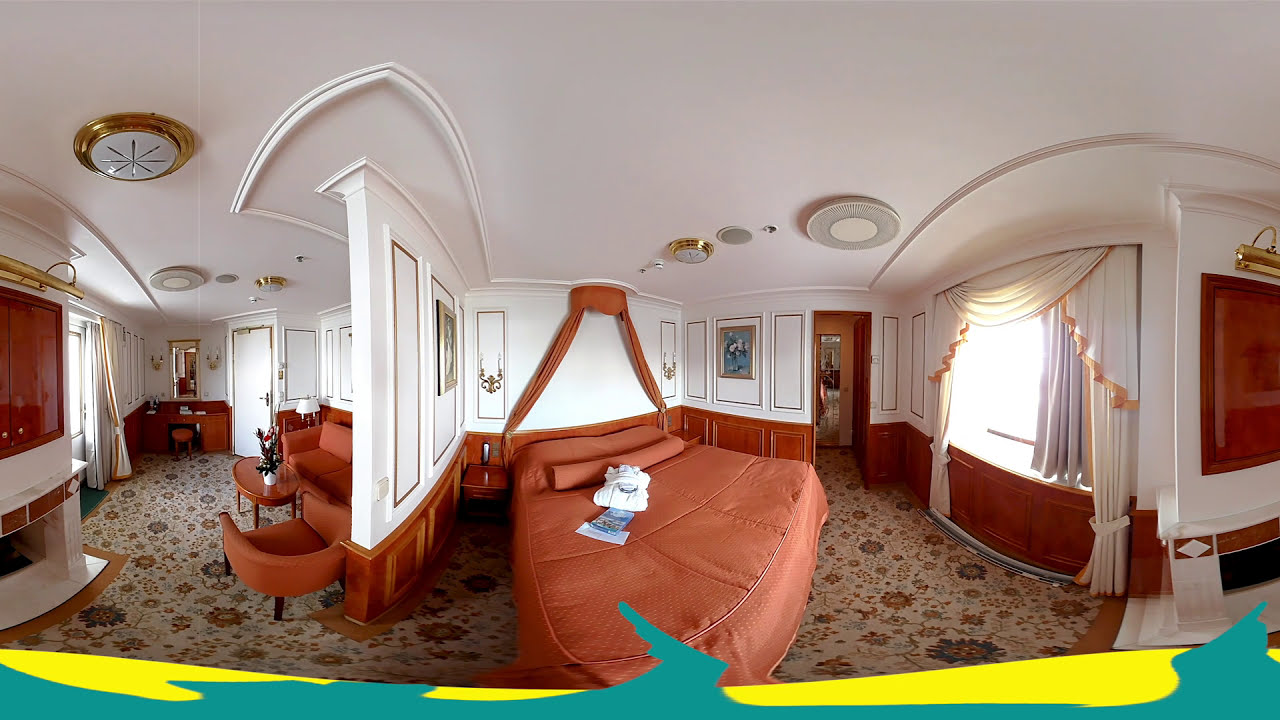The image captures an intricately designed bedroom, likely taken with an extreme wide-angle lens, giving the room a distorted, curved appearance. Dominating the center is a large bed adorned with a rust orange comforter and matching pillows, complemented by carefully folded white towels. Above the bed, a drape in a matching rust shade is elegantly arranged in a triangular shape. The room's floor features a floral pattern, adding a touch of sophistication.

To the left of the bed, a partial wall divides the room, revealing a sitting area with a matching rust orange couch and armchair, beside a white marble fireplace. The walls of the room are ornate, with dark brown wood trim along the bottom and golden rectangular frames embellishing the upper sections. Some of these frames contain paintings and candlestick-like light fixtures. Golden-edged curtains frame a window thoughtfully draped beside the bed. A desk with a small stool is positioned against the back wall, alongside the entry door, completing the opulent look of this bedroom or hotel room.